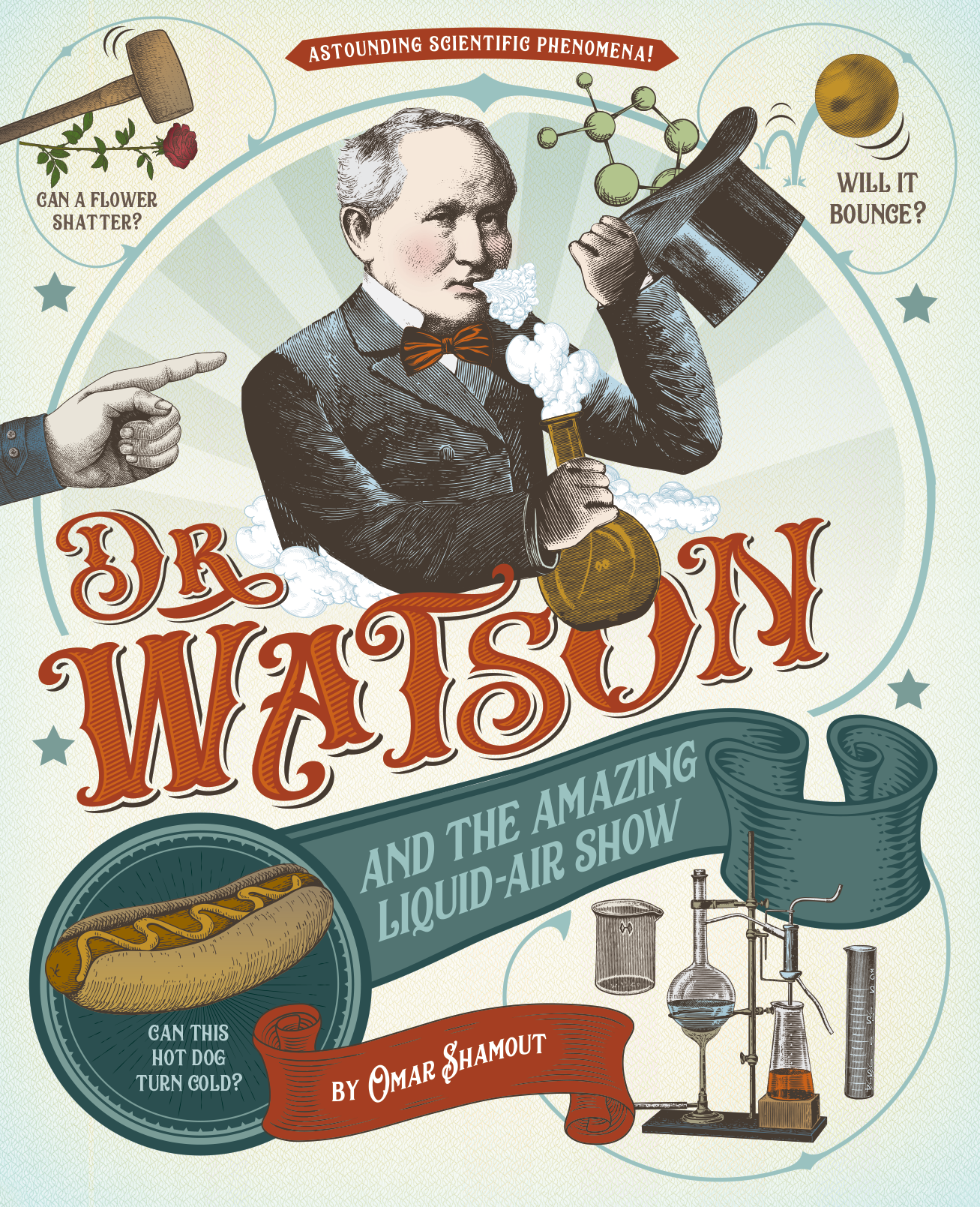An advertisement styled from the late 1800s to early 1900s showcases "Dr. Watson and the Amazing Liquid Air Show" by Omar Shamoud. In a vertically aligned rectangle, the eye is drawn to the upper center, where a man in a black suit jacket and red bow tie stands prominently. He holds a flask emitting white smoke in his right hand, while his left hand clutches a black top hat. Above him, a red banner with white letters proclaims "Astounding Scientific Phenomena!" 

Green and orange accents highlight key elements such as the green banner reading "Amazing Liquid Air Show," and the large, curvy orange letters spelling out "Dr. Watson." Surrounding the main figure, colorful vignettes illustrate various "scientific" marvels: the upper left corner depicts a hammer poised to strike a flower, above the caption "Can a flower shatter?" The upper right corner shows a gold ball accompanied by the question, "Will it bounce?" In the lower right, an array of test tubes and beakers is displayed.

Below the central man, an image of a hot dog is accompanied by the phrase, "Can this hot dog turn cold?" Across the bottom, a banner in white letters credits Omar Shamoud. The background is a vibrant mix of green, blue, white, yellow, orange, and black, evoking a sense of the traveling medicine shows and their often-questionable scientific exhibitions.